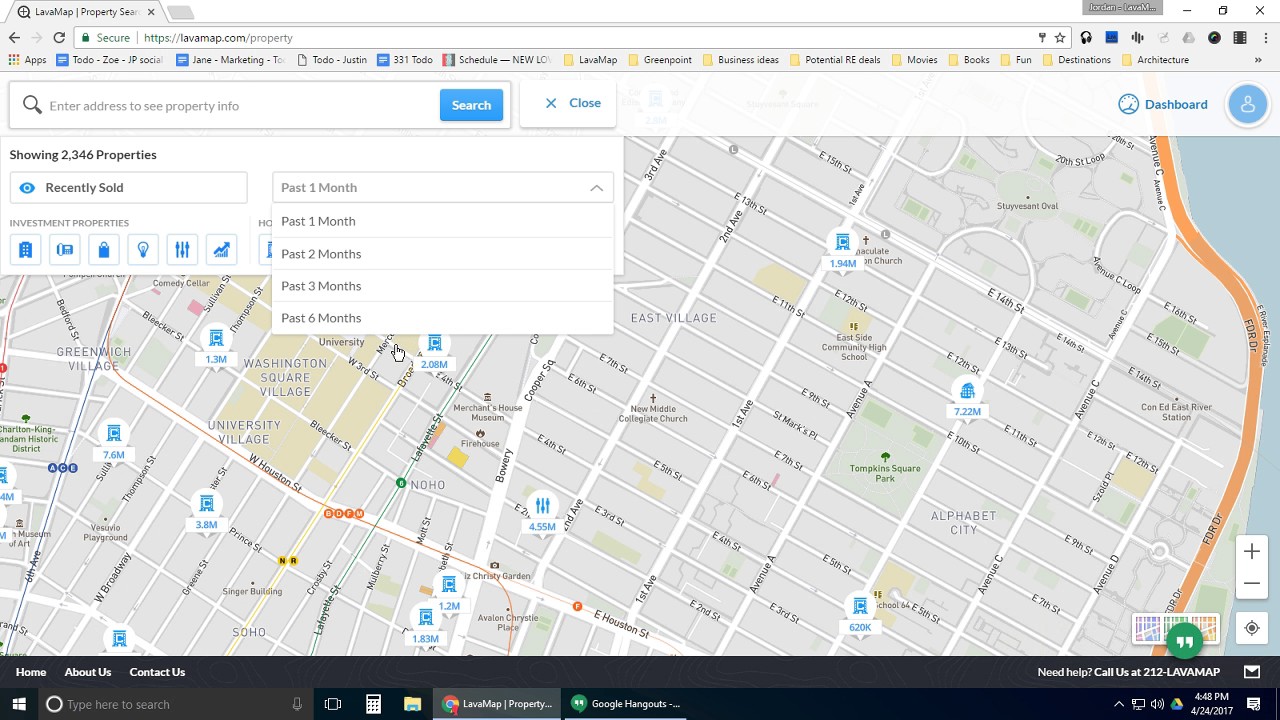The image captures a web browser displaying the LavaMap website, specifically on the 'Property' page, as shown by the URL: lavamap.com/property. The bookmark bar below the URL box features an array of bookmarks titled: Apps, Toto, Zoe, Jane Marketing, Toto, Justin, 331 Toto, Schedule, New, LavaMap, Greenpoint, Business Ideas, Potential, RE Deals, Movies, Books, Fund, Destination, Architecture.

Centered on the page is a search box prompting users to "enter address to see property info," accompanied by a blue 'Search' button and options labeled 'Close' and 'Dashboard.' Just beneath this input field, a status line indicates, "Showing 2,346 properties recently sold past one month."

Highlighted on the map are pin locations for various places including the East Village, Washington Square Village, and Greenwich Village, effectively marking recently sold properties within these neighborhoods.